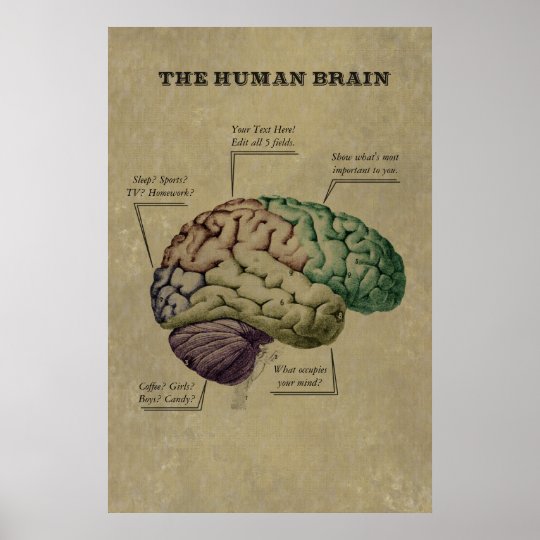The image showcases a vintage, beige piece of paper with "THE HUMAN BRAIN" typed in all capital letters at the top in a serif font. Centered on the paper is an illustration of a brain, presented in a side view and segmented into various colors. These colors include purple at the bottom, a dirty olive beige in the middle, brown towards the top, and green at the very right-top side. Each section of the brain is labeled with different captions: the green part reads "Show what's most important to you," the brown section is marked "Your text here, edit all five fields," and the purple part includes "Sleep, sports, TV, homework." Additionally, the lower purple section is labeled with "Coffee, girls, boys, candy." At the bottom of the paper, there is a question, "What occupies your mind?" followed by a question mark. The brain's vibrant color scheme contrasts with the antique appearance of the page, giving it an instructional and reflective feel.